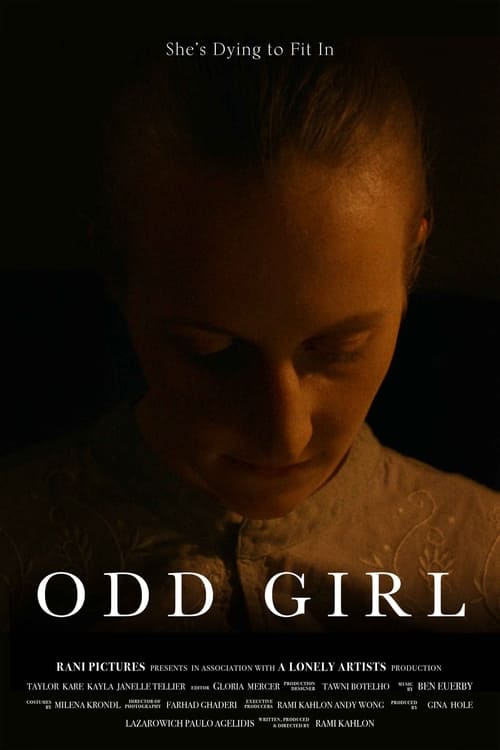This is a detailed movie poster for the film "Odd Girl." The upper portion of the poster features the slogan "She's dying to fit in" written in white text against a dark background. Dominating three-fourths of the image is a photograph of a girl with a pale complexion, expressionless face, and her hair pulled back behind her ears. Her head is bowed, eyes cast downwards, casting her face in partial shadow. She wears a white lace shirt with black detailing that extends up to her neck, resembling a half-neck style. The title "Odd Girl" appears near the bottom in prominent white text, followed by the credits, which read "Rani Pictures presents in association with a Lonely Artist production," and additional smaller text. The overall background of the poster is black, creating a stark contrast with the white text and the girl's image.